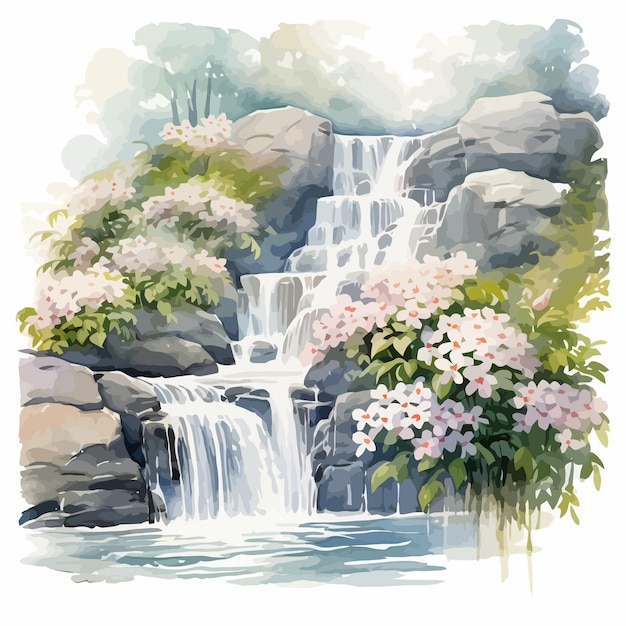The image is a detailed artistic representation of a cascading waterfall flowing down a series of gray rocks. The waterfall, depicted almost in a watercolor style, appears to start at the top left and flows towards the right, descending in stages. At the base, the water collects into a shallow, slightly blue pool. On either side of the waterfall, there's lush green vegetation, adorned with patches of pink flowers, possibly growing out of the moss on the rocks. White flowers with orange centers are also visible. At the top of the image, slightly washed out trees, with the sun shining through them, give a serene backdrop to the vibrant foreground. The clean, digitally-rendered look of the image suggests it might be computer-generated, emphasizing clear, distinct shapes and colors, capturing an aesthetic reminiscent of Asian art.